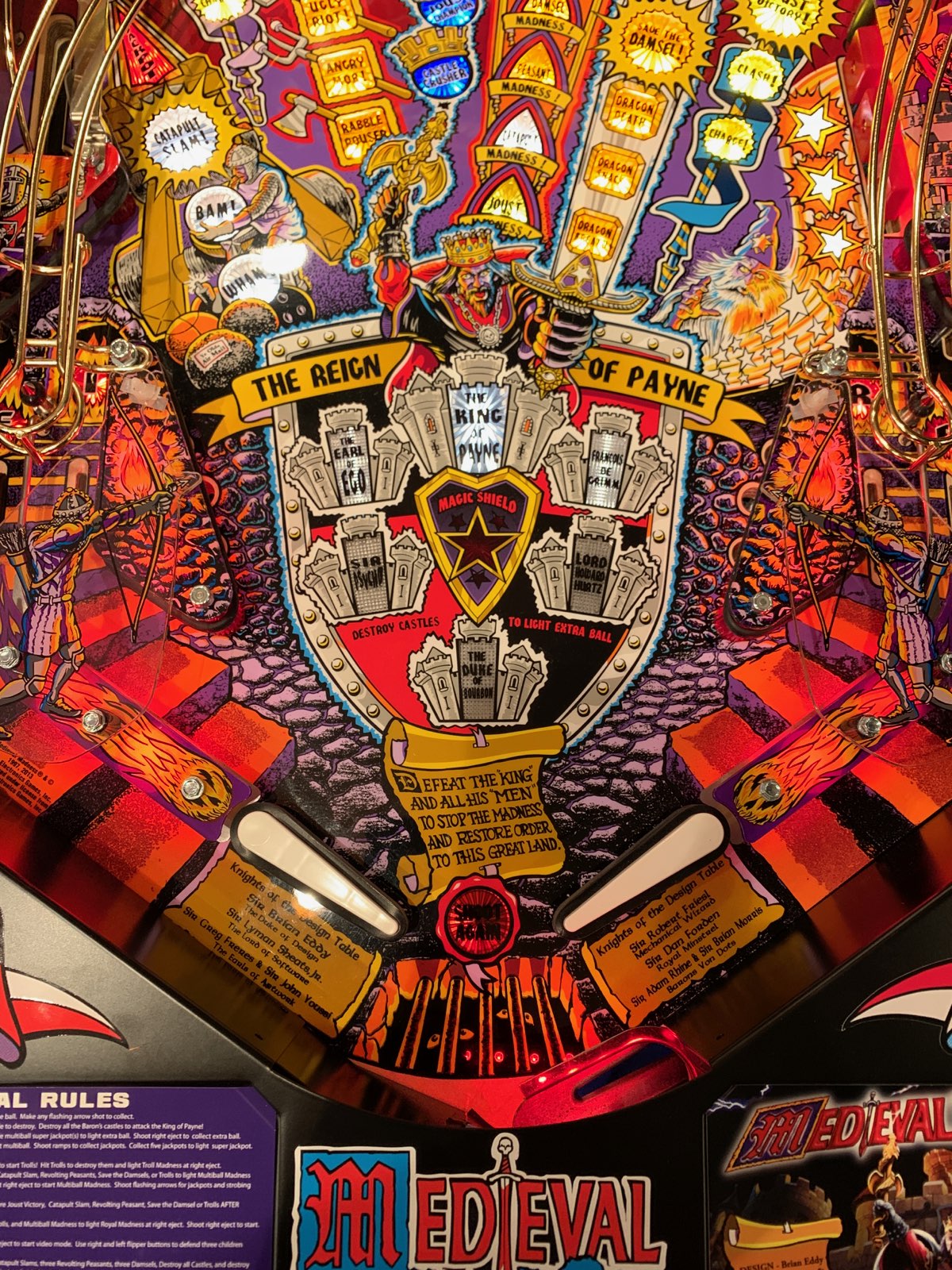The image depicts a medieval-themed slot machine or pinball machine adorned with vivid yellows, reds, and blues. The bottom of the machine prominently features the word "MEDIEVAL" in large, red calligraphy-style letters on a blue background, with a sword ingeniously incorporated as the 'I' in "MEDIEVAL". Rules of the game are clearly shown on a purple background with white text to the left side of the image. Above it, various sections of the game display detailed artwork, including a fearsome king holding a scepter and a large sword. The game, titled "The Reign of Pain," includes phrases such as "The Reign of Pain", "The King of Pain", "Magic Shield", "The Earl of Ego", and "Destroy Castles to Light Extra Ball". Additional game features include a crest in black and red, depicting castles and smaller intricate designs with small text. The machine includes visible gold rails and white flippers, contributing to its rich, detailed medieval aesthetic.